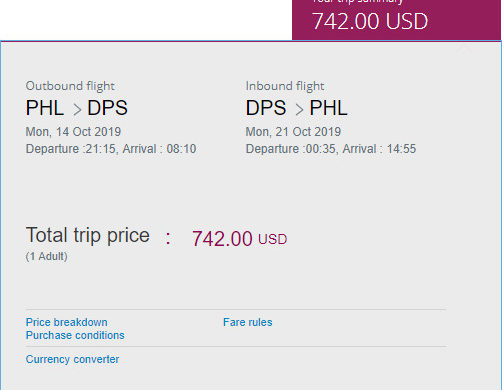In this screenshot, we see a large square bordered by thin purple lines at the top and thin blue lines on each side. The interior of the square is light gray. Prominently displayed is a magenta pink rectangle with white text, indicating a total trip price of $742.

The details of the trip are clearly outlined:

- **Outbound Flight**: Originating from Philadelphia International Airport (PHL) with an arrow pointing to Ngurah Rai International Airport (DPS). Departure is scheduled for Monday, October 19th at 21:15, with arrival at 08:10.
- **Inbound Flight**: From Ngurah Rai International Airport (DPS) returning to Philadelphia International Airport (PHL). Departure is on Monday, October 21st at 00:35, arriving at 14:55.

This information is written in black text, while the total trip price of $742 is emphasized in magenta pink. The fare is for one adult.

Below this information, there is a gray horizontal line. Underneath, in blue text, are links labeled “Price Breakdown,” “Purchase Conditions,” and “Fare Rules.” Another line follows, leading to a “Currency Converter” option.

Overall, the layout is clean and well-organized, with key details highlighted for easy reference.